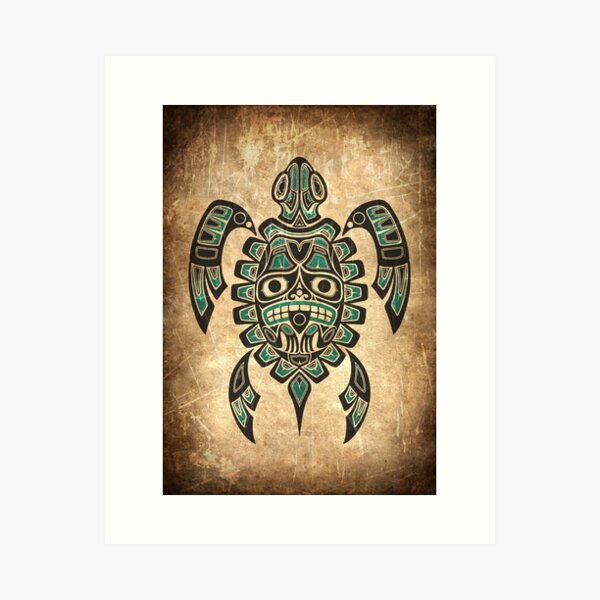The image is a detailed, indigenous-style illustration of a sea turtle, evocative of Pacific Northwest or Alaskan Native American art. The turtle's carapace features a central human warrior face with large black eyes, large teeth, and a spade-shaped nose. On the turtle's stomach, the illustration continues with two hands below the face, each with three fingers and green plates on top. Below the hands is a shield, flanked by two triangular shapes, and the turtle's tail features a green heart bordered in black, tapering to a sharp point. The front flippers are artistically rendered to resemble birds, with what appear to be bird's eyes and beaks at the point where the flippers join the carapace. The rear flippers share a similar style but are less distinctly bird-like. The entire piece is rendered in dark brown with turquoise and cream accents and is set against a light brown background with darker, vignetted corners that give the impression of aged papyrus or bark. The artwork is framed in white, enhancing the indigenous aesthetic.